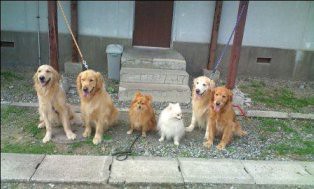A photograph captures six dogs sitting obediently in a line on a rocky, grassy ground, positioned between a small concrete sidewalk and a set of three cement steps. The steps lead up to a dark brown, partially visible door flanked by four mahogany-colored poles to which the dogs' leashes are attached. The dogs on either end are large, fluffy golden retrievers with their leashes secured to the poles behind them. In the center are two tiny, fluffy Pomeranian puppies, one tan and one white, both with leashes hanging loosely. Adjacent to the center Pomeranians are two more golden retrievers, one tan and one darker brown. All the dogs, except the small white Pomeranian which gazes off to the side, face forward with calm, content expressions. Behind the dogs, the building has white plaster walls with a dark gray lower section, an industrial appearance, and a gray trash can beside the steps. The area in which the dogs sit exhibits patches of scrubby grass amidst the gravel.